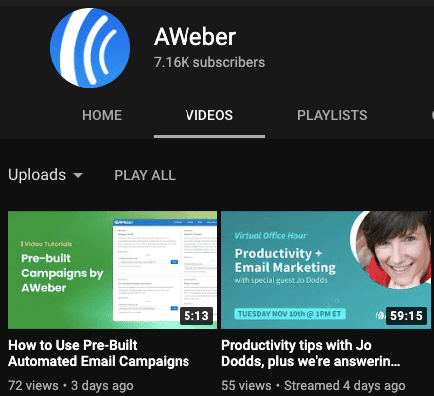The image depicts a section of a computer screen showcasing a YouTube channel titled "A. Weber." Adjacent to the title is a blue circle emblem featuring three curved white stripes. The channel boasts 7.16 thousand subscribers. 

Centered horizontally across the page are three navigation tabs in white capital letters: "HOME," "VIDEOS," and "PLAYLISTS." The "VIDEOS" tab is distinctly highlighted in a brighter white and underlined, indicating the current active page. The page background is black, providing a stark contrast to the text.

Directly below the navigation tabs, a section labeled "Uploads" is visible, featuring a "Play All" button. Two video thumbnails are displayed side by side; the left thumbnail with a green background and the right with a blue background labeled "Product Productivity and Email Marketing." The green thumbnail showcases a video titled "Pre-Built Campaigns by A. Weber," while both thumbnails include video durations and detailed descriptions below.

The first video, "How to Use Pre-built Automated Email Campaigns," has gathered 72 views within three days of uploading.